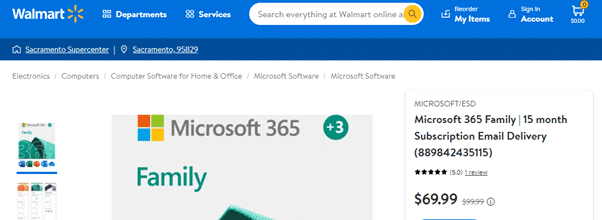A partial screenshot of a Walmart web page features a prominent blue banner at the top. On the banner's top left, the word "Walmart" is displayed in white along with the company's distinctive orange burst logo, which resembles a flower without a stem. The banner also includes white text for "Departments" and "Services," a long white oval search bar, and icons for "My Home," "Account," and "Cart," the latter of which shows an orange circle with a zero, indicating an empty cart.

Below the banner, the page is partially visible, showcasing a product listing for "Microsoft 365." The Microsoft logo, consisting of four colored squares (red, green, blue, and orange) arranged in a grid pattern, accompanies the product title "Microsoft 365." Adjacent to this, a green circle with white text says "plus 3," followed by the word "Family" in the same green color. A fragmented image appears below this text, only partially visible, revealing the top of a triangular shape. To the left, a smaller version of this page is partially visible, along with some blurry text.

To the right, detailed product information is provided, stating "Microsoft / ESD, Microsoft 365 Family, 15 Month Subscription, Email Delivery." The listing also includes an item number, a 5-star rating based on one review, and a sale price of $69.99, down from the original price of $99.99, which is crossed out and presented in smaller, unbolded text.